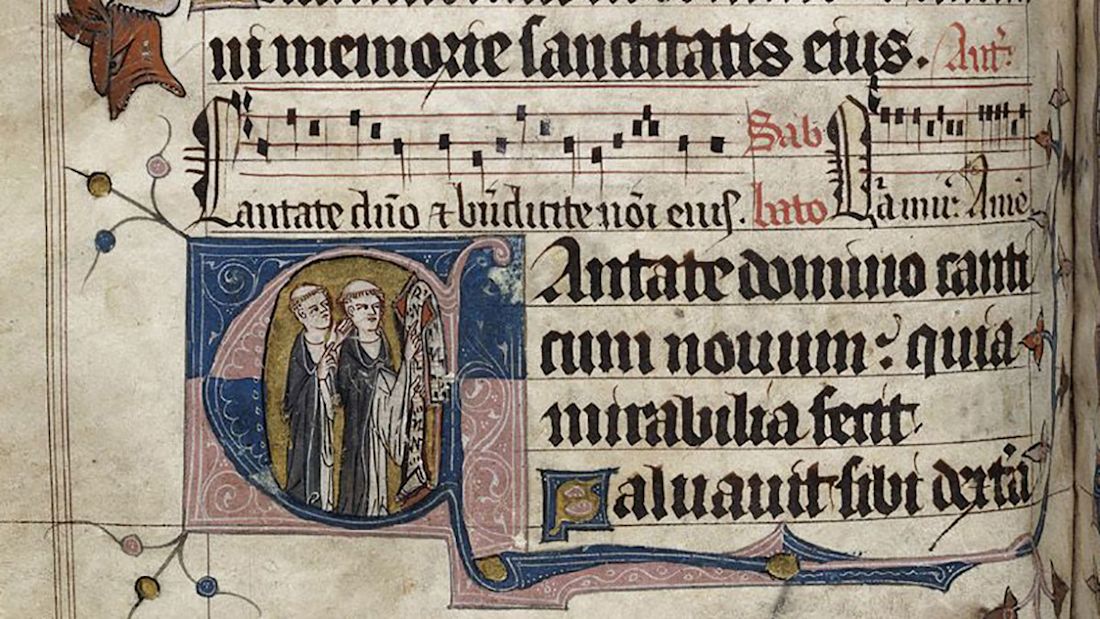This detailed photograph captures an ancient medieval manuscript, likely a hymn book, featuring a blend of ornate calligraphy, musical notation, and vivid illustrations on a white-grayish background. The page, part of an open book presented in landscape orientation, displays a richness of historical detail.

At the top left corner, there's a striking, hand-drawn head of a cat or fox facing downward, possibly in distress. This is followed by large, bold calligraphy in Latin. Below the text, a line of meticulously rendered music notes on a scale, or stave, hints at the book’s musical nature.

Further down, the manuscript displays another block of text in Latin, succeeded by a colorful illustration. This illustration depicts two monk-like figures with traditional tonsured hairstyles, dressed in blue robes, examining a scroll together. They are framed within a blue and pink ornamental border situated at the bottom left of the page. Surrounding this illustration, additional Latin text is arranged, intermixed with more sections of musical notation.

The entire composition, with its six lines of text and one line of musical notation, encapsulates the religious and artistic heritage of the medieval period, revealing a vivid snapshot of history through its hand-drawn and hand-written elements.